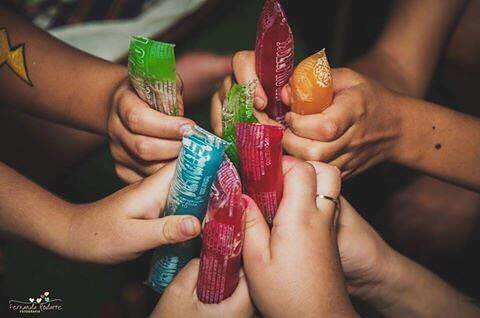This semi-professional photograph captures a vibrant display of seven children's hands, each grasping colorful frozen Icy Pops of various flavors. The hands, adorned with distinct features such as nail polish, a ring, black moles, and a temporary lightning bolt tattoo, converge in the center of the image, seemingly in a celebratory toast. The frozen treats vary in flavor, presenting a playful spectrum of green, blue, red, orange, and purple hues. The blurred white background and barely visible writing in the lower left-hand corner add a touch of mystery, while the composition emphasizes the carefree spirit of the scene, suggested by the children's bare, sleeveless arms.